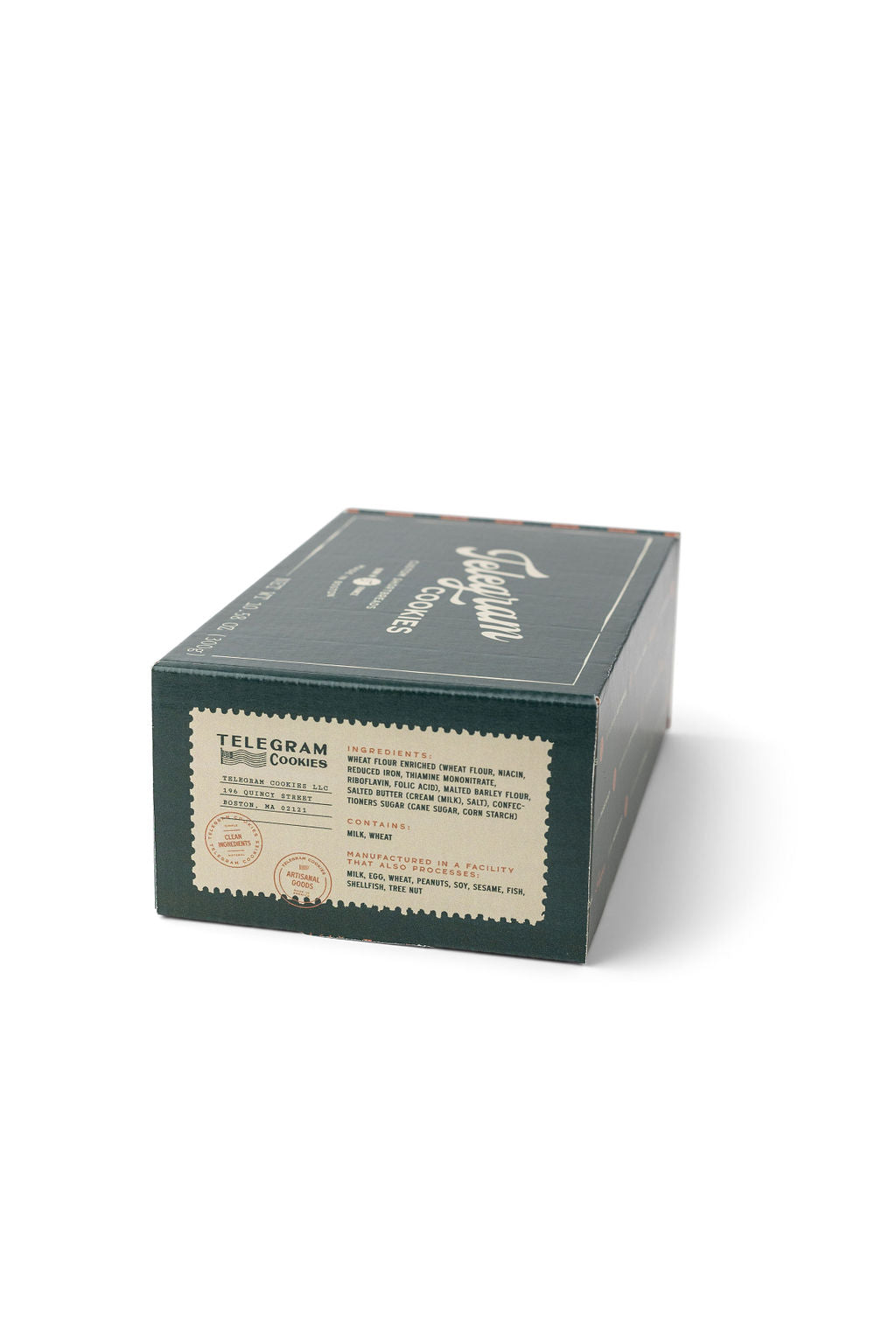The image features a small, dark green cardboard box with a swivel top lid, designed similarly to a shoe box in shape and size, approximately three inches by two inches. The box prominently displays the brand name "Telegram Cookies" in a cursive font on the top, though the text appears slightly blurry. The side of the box is the focal point of the image, providing crucial details including an address indicating the cookies are from Boston, Massachusetts. The side also features an illustration of a long American flag and two red stamp-like images that read "clean ingredients" and "artisanal goods." The box lists comprehensive ingredients such as enriched wheat flour, malted barley flour, buttercream, confectioner's sugar, cane sugar, and corn starch. It also includes a warning that the cookies contain milk and wheat, and were manufactured in a facility that processes several allergens including milk, egg, wheat, peanuts, soy, sesame, fish, seashells, and tree nuts.